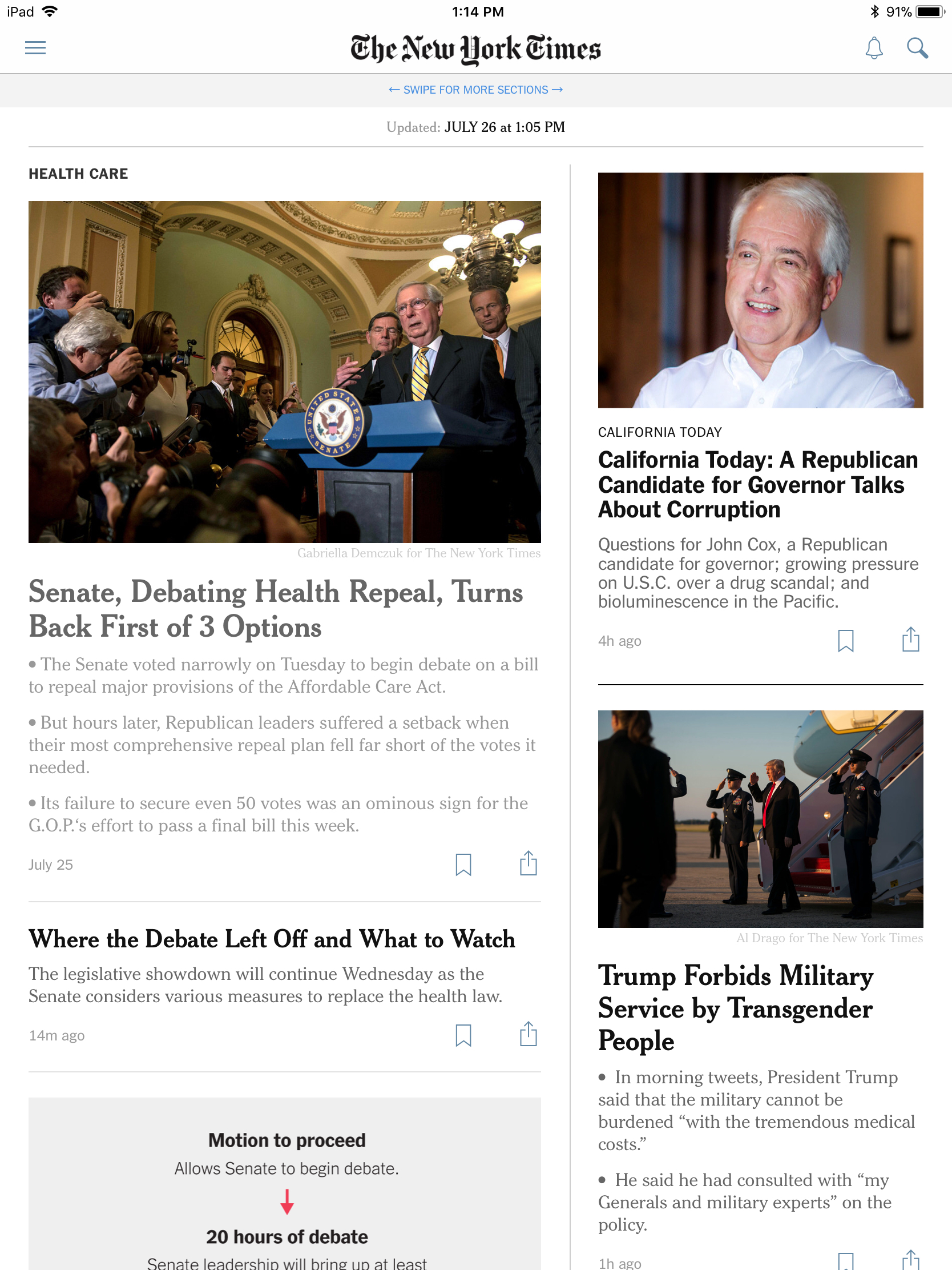In this screenshot of The New York Times, dated July 26th, the primary focus is a photograph featuring Senator Mitch McConnell standing at a podium, delivering a speech amidst an array of photographers and journalists. The accompanying headline reads: "Senate Debating Health Repeal Turns Back Five of Three Options."

The article details how the Senate narrowly voted on Tuesday to begin the debate on a bill aimed at repealing key provisions of the Affordable Care Act. Despite this initial progress, Republican leaders encountered a significant setback as their most comprehensive repeal plan failed to secure even 50 votes, signaling potential challenges for the GOP's efforts to pass final legislation within the week. The piece also highlights an upcoming legislative showdown set for Wednesday, during which the Senate would consider various alternative measures to replace the existing health law.

Additionally, the screenshot includes snippets from other articles:
- "California Today" covers a Republican gubernatorial candidate discussing corruption and featuring a Q&A with John Cox, another Republican candidate for governor.
- There is growing pressure on the University of Southern California (USC) in relation to a drug scandal.
- An article also mentions bioluminescence in the Pacific.

Further down, another headline reads: "Trump Forbids Military Service by Transgender People." This section explains that in a series of morning tweets, President Donald Trump announced that transgender individuals would be prohibited from serving in the military, citing consultations with his generals and military experts, and the “tremendous medical costs” involved. This snapshot captures a significant moment in contemporary politics, particularly concerning healthcare and civil rights.